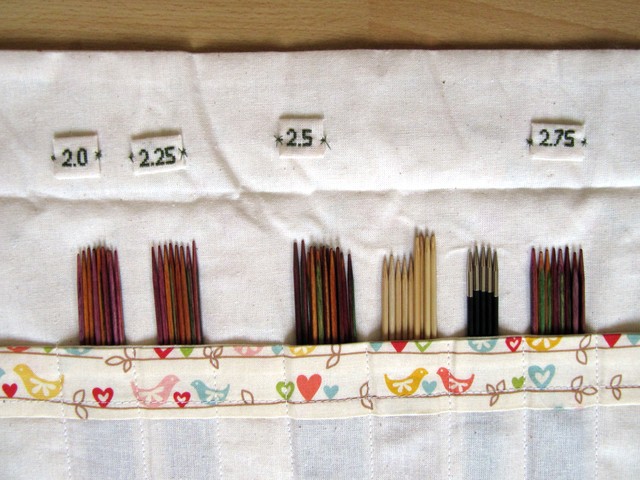This image features a handmade, white fabric pouch designed specifically for organizing knitting needles, neatly displayed on a laminate wood grain surface. The pouch has a fold-over top and is divided into several stitched pockets, each labeled with needle sizes: 2.0, 2.25, 2.5, and 2.75 millimeters. The various knitting needles range in color from a dark reddish-brown, black, and bronze to a natural blonde wood. Each section is meticulously stitched to securely hold the needles. A decorative embroidered trim runs along the bottom of the pouch, adorned with images of small doves, hearts, and various leaf designs in subdued hues of pale purple, amber, and green.